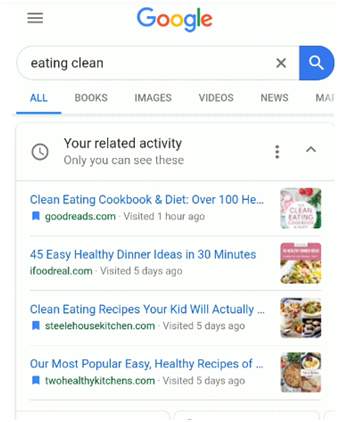The image is a screen capture from a Google search interface. The background is predominantly white, with the colorful Google logo prominently displayed at the center top. Below the logo is the search bar, which has a white background and contains the text "eating clean" in black font. On the far right of the search bar is an 'X' icon. Adjacent to the search bar is a blue button shaped like a half-circle with a white magnifying glass icon inside it.

Directly underneath the search bar is the navigation panel with sections labeled from left to right: All, Books, Images, Videos, News, and a partially visible 'More'. Below this panel are the search results for "eating clean," featuring relevant books and articles.

The first section displays the message "Your related activity," followed by "Only you can see these" in black text. There are four search results, each highlighted in blue:

1. "Clean Eating Cookbook and Diet: Over 100 HE..." 
2. "45 Easy Healthy Dinner Ideas in 30 Minutes"
3. "Clean Eating Recipes Your Kid Will Actually..."
4. "Our Most Popular Easy Healthy Recipes of..."

These results link to four respective websites: Goodeats.com, Ifoodreal.com, Steelhousekitchen.com, and Twohealthykitchens.com, each accompanied by a small icon representing the website or book to the right of the search result.